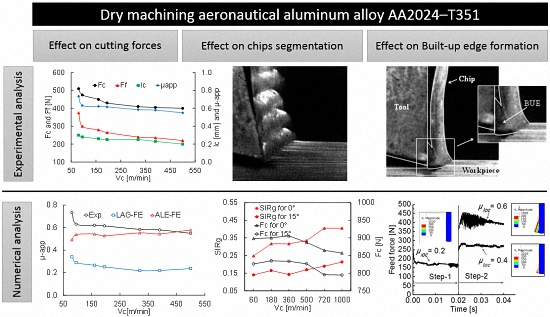The image is a detailed technical sheet you might encounter online or in a specialized technical magazine or book. At the top of the image in a black bar with white text, the title reads "Dry Machining Aeronautical Aluminum Alloy AA2024-T351." Beneath this header, three grey rectangles provide further insight, stating in black text: "Effect on Cutting Forces," "Effect on Chip Segmentation," and "Effect on Built-Up Edge Formation." 

The central section features an array of detailed diagrams. The top row includes a chart to the left with a multi-colored line graph featuring green, red, blue, and black lines plotting data on the X and Y axes. To the right of this are black-and-white photographs; the first depicts four spherical objects, potentially reflective of the tested materials, and the second image shows what looks like an annotated depiction of machining elements with labels such as "Tool," "Chip," "Workpiece," and "BUE" (Built-Up Edge).

The lower section of the image is dominated by more analytical charts and graphs. On the far left, two grey rectangles run vertically, labeled "Numerical Analysis" at the bottom left corner and "Experimental Analysis" immediately above. Other graphs depict lines in various colors, including black, red, and blue. One graph in the middle features two red and two black lines, while another on the bottom right corner shows three squiggly black lines, underscored by a legend featuring colors like red, orange, yellow, green, and blue. Additional annotations include mentions of "feed force" and "time," tying into the experimental data presented.